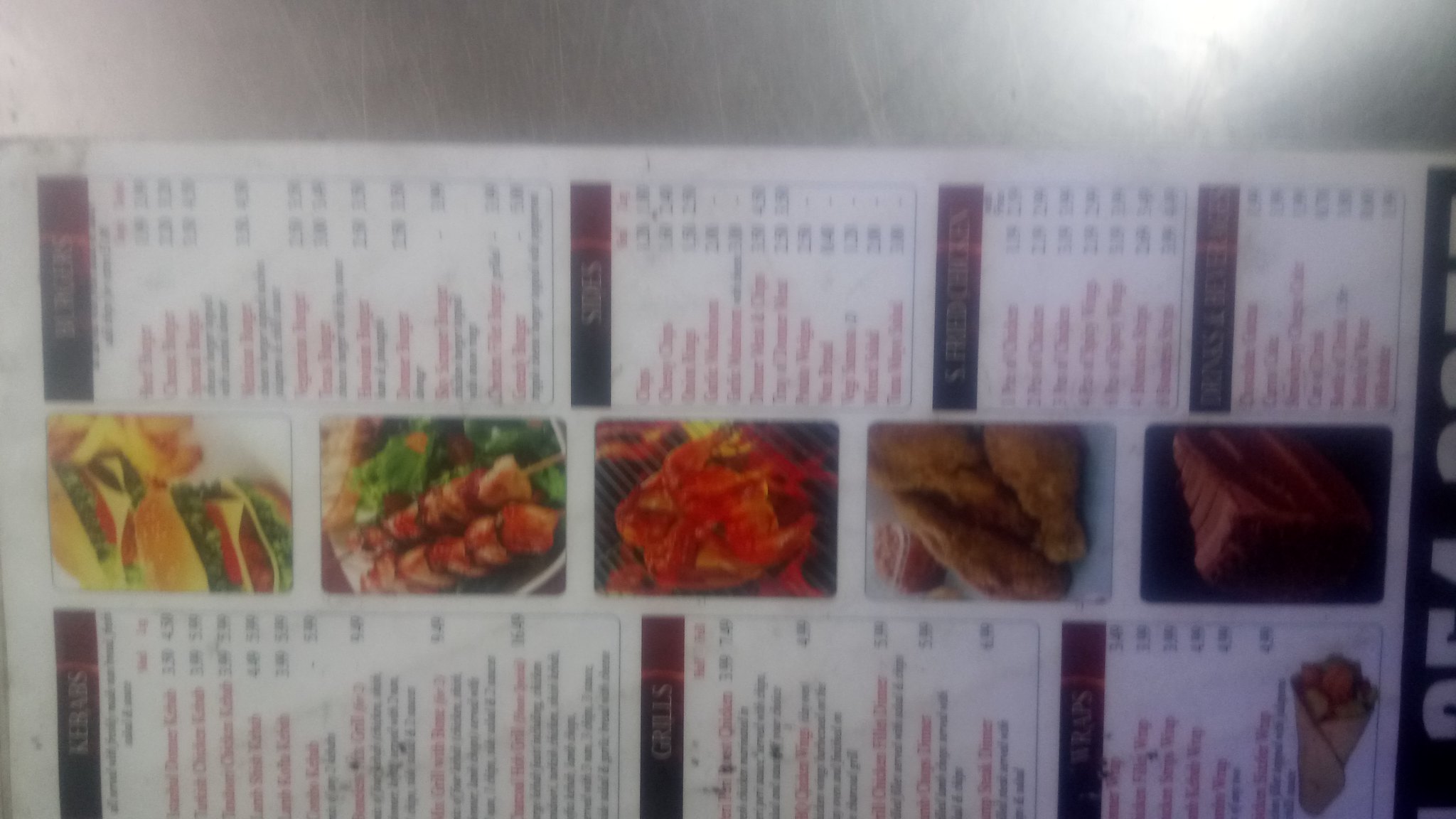The image is a photograph of a sideways menu, requiring viewers to rotate their computer to read it properly. The menu is divided into three vertical sections: the left and right sides contain menu items, while the center is filled with images of various dishes, making them the focal point. 

From the top, the first picture showcases two cheeseburgers accompanied by a side of French fries. Below it is an image of kebabs, featuring skewered meat arranged on a bed of lettuce with some unidentifiable, slightly blurred components. Continuing downward, the next picture is ambiguous but suggests a possible seafood dish. Further down, a clear image of fried chicken is displayed. The final picture at the bottom of the column tantalizes the viewer with a piece of chocolate cake, lavishly covered in chocolate icing.

Readable headings on the menu include "Kebabs," "Grills," "Sides," and "S Fried Chicken," which likely refers to Southern Fried Chicken. However, several other headings remain unreadable.